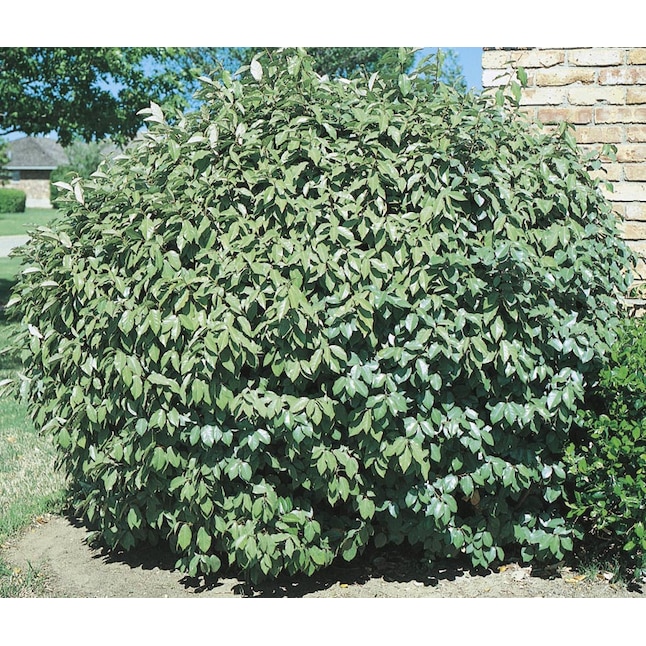The photograph showcases a tall, wide, and lush green bush, likely a butterfly bush, positioned outside a reddish-brown brick house. This prominently large bush, estimated to be about three to four feet tall, is entirely covered with over 200 narrow, pointed leaves of a muted green shade, without any blossoms. Adjacent to this bush is a neatly kept, short grass lawn. In the background, a clear blue sky frames the scene, alongside a partial view of the house's brick wall and several other houses, including one across the street adorned with shrubs. Surrounding trees add depth to the scene, indicating a spring setting with greenery beginning to flourish, albeit sporadically dotted with brown patches from drought-resistant Bermuda grass.